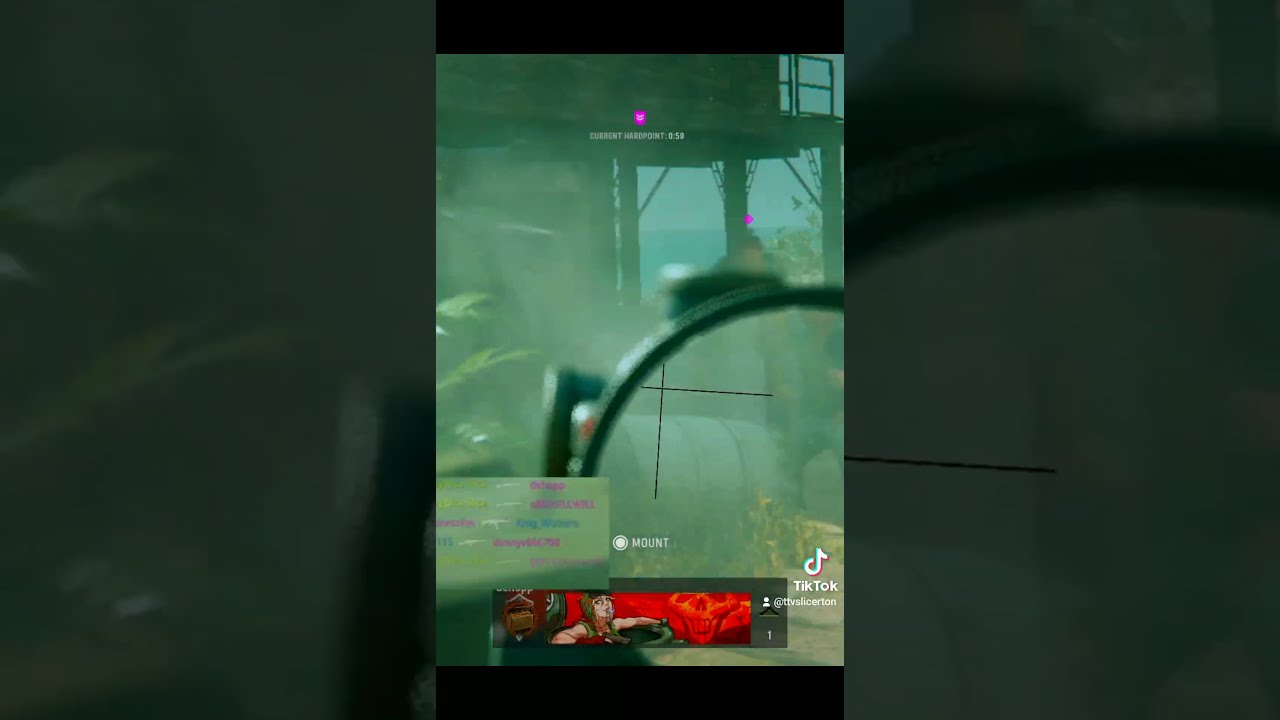The image is a screenshot, likely taken from TikTok or another social media platform like Instagram Live, which features a still from a first-person shooter game. The central focus of the image includes the crosshairs of a gun's scope positioned towards the bottom right. The backdrop appears to be a war zone depicted with various colors: gray, green, black, white, red, purple, pink. Notably, the bottom part of the screen has a green rectangle serving as a banner that houses different visual elements. Within this green banner, there's a red skull next to a character, likely a woman, against a red background. Additionally, the text "mount" appears towards the bottom with a circle to its left. The TikTok logo is also visible in the bottom right corner, indicating the platform of origin for this screenshot.